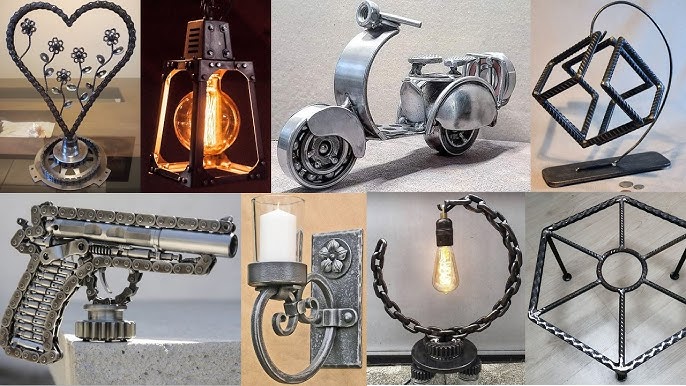The image displays an array of eight intricately designed, metal sculptures, arranged in two rows. In the top left of the first row, there's a heart-shaped piece crafted from silver metal, containing five flowers inside its frame. Following this, there's a sequence of objects including a lantern-like light fixture, a motorized bike resembling a moped, and a piece featuring interconnected squares. In the bottom row, the first image shows a sectional view of a metallic gun, revealing the internal bullets lined up neatly in its handle. Alongside these, there's another light fixture designed for a candle, a light bulb holder, and a sculpture that resembles a small table. Many of these sculptures appear to be built from parts of a sewing machine, giving them a custom, repurposed aesthetic.